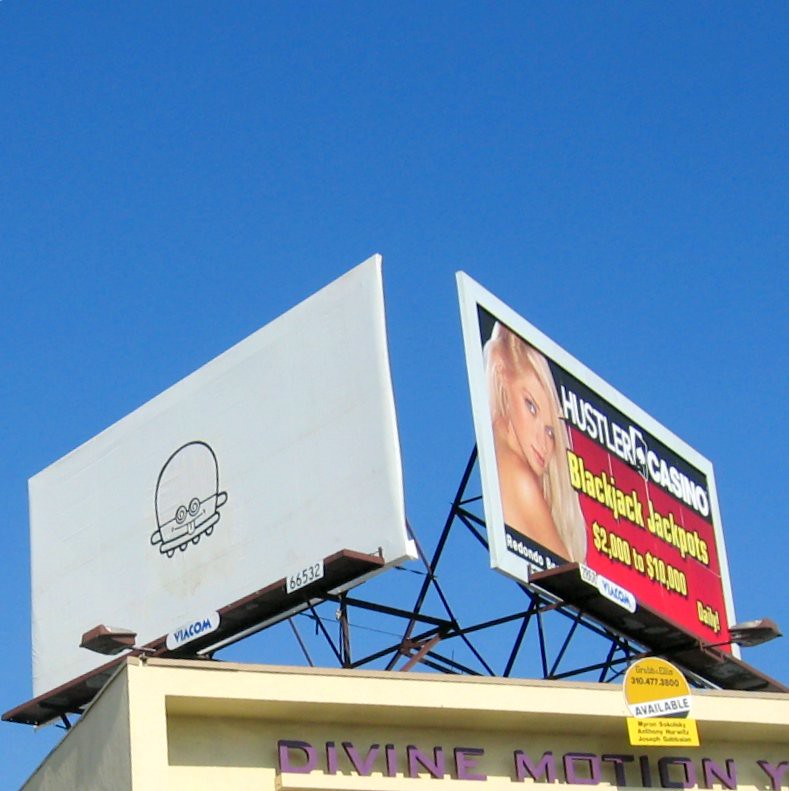The image is an outdoor scene set against a clear blue sky. On the left side of the image, there is a white billboard. At the center of this billboard, there is an illustration resembling a rounded head with two eyes and a tongue sticking out; beneath this head-like figure are several round shapes and four smaller circles, suggesting a UFO-like appearance but focusing on the head. The billboard is branded with "Viacom." The number "66532" is also visible on this billboard.

On the right side of the image, there is another billboard advertising Hustler's Casino. This billboard has a prominent red square background with yellow text that reads, "Blackjack Jackpots $1,000 to $10,000 Daily." To the left of this main text is the image of a blonde woman framed by a white background. At the very bottom of this billboard, the words "Divine Motion" are displayed in purple text. Below this, there is a yellow circle with black text featuring a white slash, followed by another yellow sign.